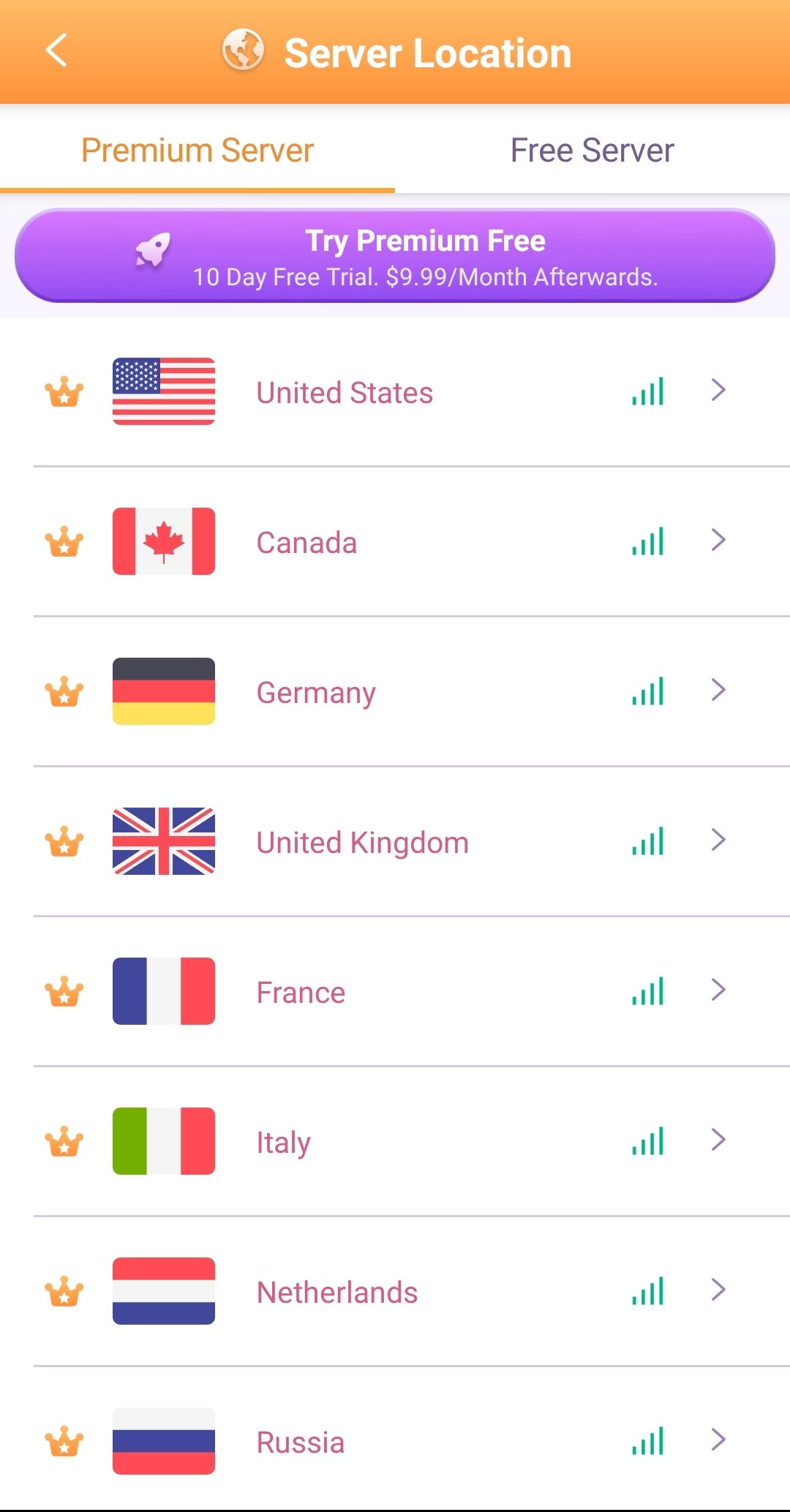This screenshot from a smartphone displays a webpage with a focus on server location options for a VPN service. 

**Description:**

At the top of the screenshot, an orange banner with a white globe icon contains the text "Server Location." To the left is a left-facing arrow for navigation. Below the banner, two tabs are visible: "Premium Server" (currently selected) and "Free Server." 

Under the tabs, a lavender-colored box with white text offers a promotional trial, stating: "Try Premium Free, Ten-day free trial, $9.99/month afterwards."

The main section of the page lists eight server location entries, denoted with crown icons (indicating premium status), country flags, country names, Wi-Fi icons, and right-facing arrows for selection. The entries are as follows:

1. Crown icon, American flag, "United States," Wi-Fi icon, right-facing arrow.
2. Crown icon, Canadian flag, "Canada," Wi-Fi icon, right-facing arrow.
3. Crown icon, German flag, "Germany," Wi-Fi icon, right-facing arrow.
4. Crown icon, United Kingdom flag, "United Kingdom," Wi-Fi icon, right-facing arrow.
5. Crown icon, French flag, "France," Wi-Fi icon, right-facing arrow.
6. Crown icon, Italian flag, "Italy," Wi-Fi icon, right-facing arrow.
7. Crown icon, Dutch flag, "Netherlands," Wi-Fi icon, right-facing arrow.
8. Crown icon, Russian flag, "Russia," Wi-Fi icon, right-facing arrow.

The layout is clean and straightforward, with emphasis on the premium server options available for users.